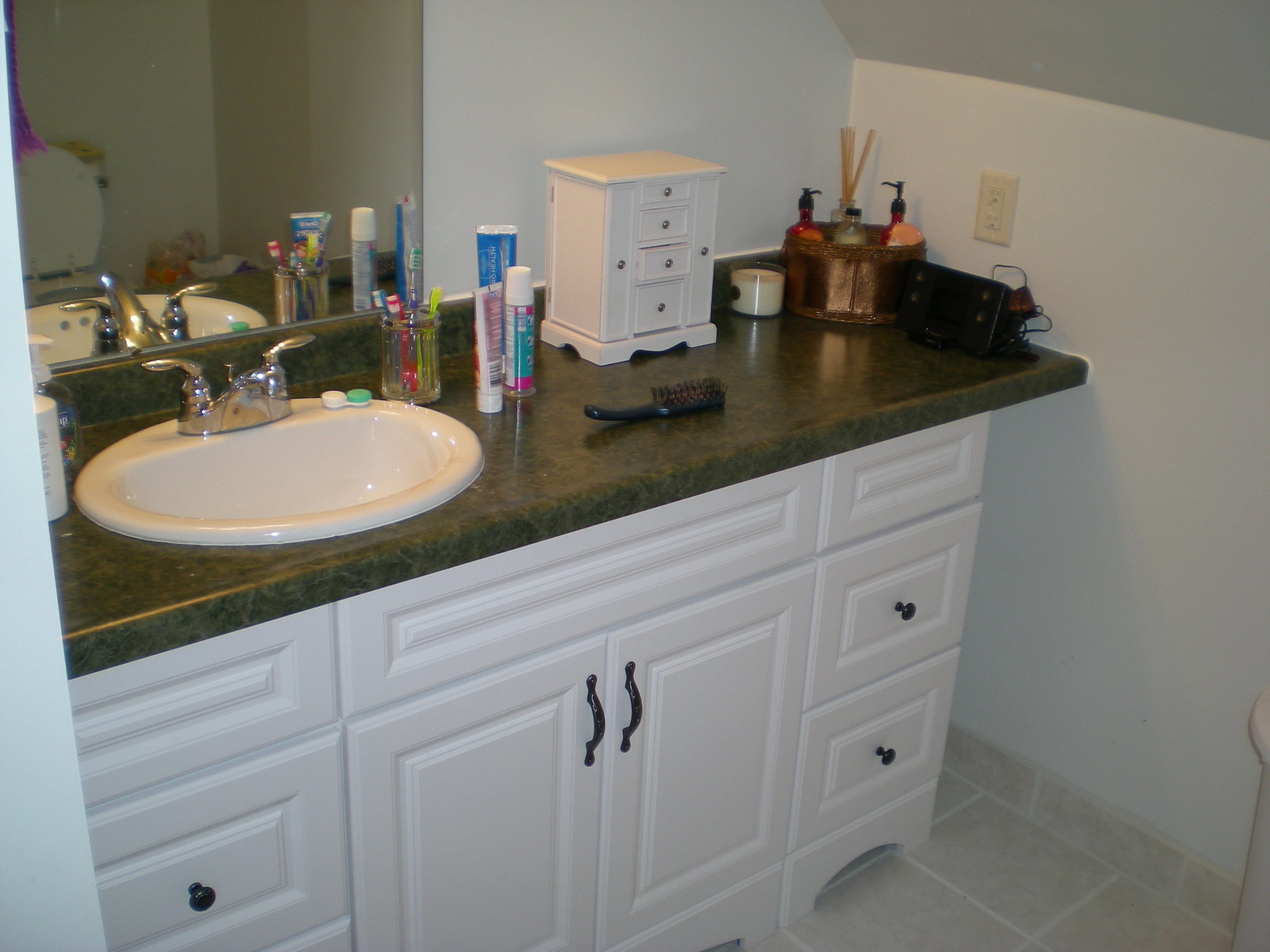This color photograph captures a contemporary bathroom with meticulous detail. At the top, a sleek mirror is prominently displayed, reflecting the modern faucet and some of the toiletries on the sink. Below the mirror, white cabinetry adorned with black handles provides a striking contrast and ample storage. The countertop features an array of everyday toiletries, including a black hairbrush, toothpaste, toothbrushes, and a hand soap dispenser. On the right side of the sink, an incense container stands adjacent to a white candle, lending a soothing ambiance to the space. Additionally, a small, white jewelry chest or set of drawers adds a touch of personal elegance. The flooring is comprised of light gray tiles with crisp white grout, completing the clean and stylish aesthetics of the bathroom.